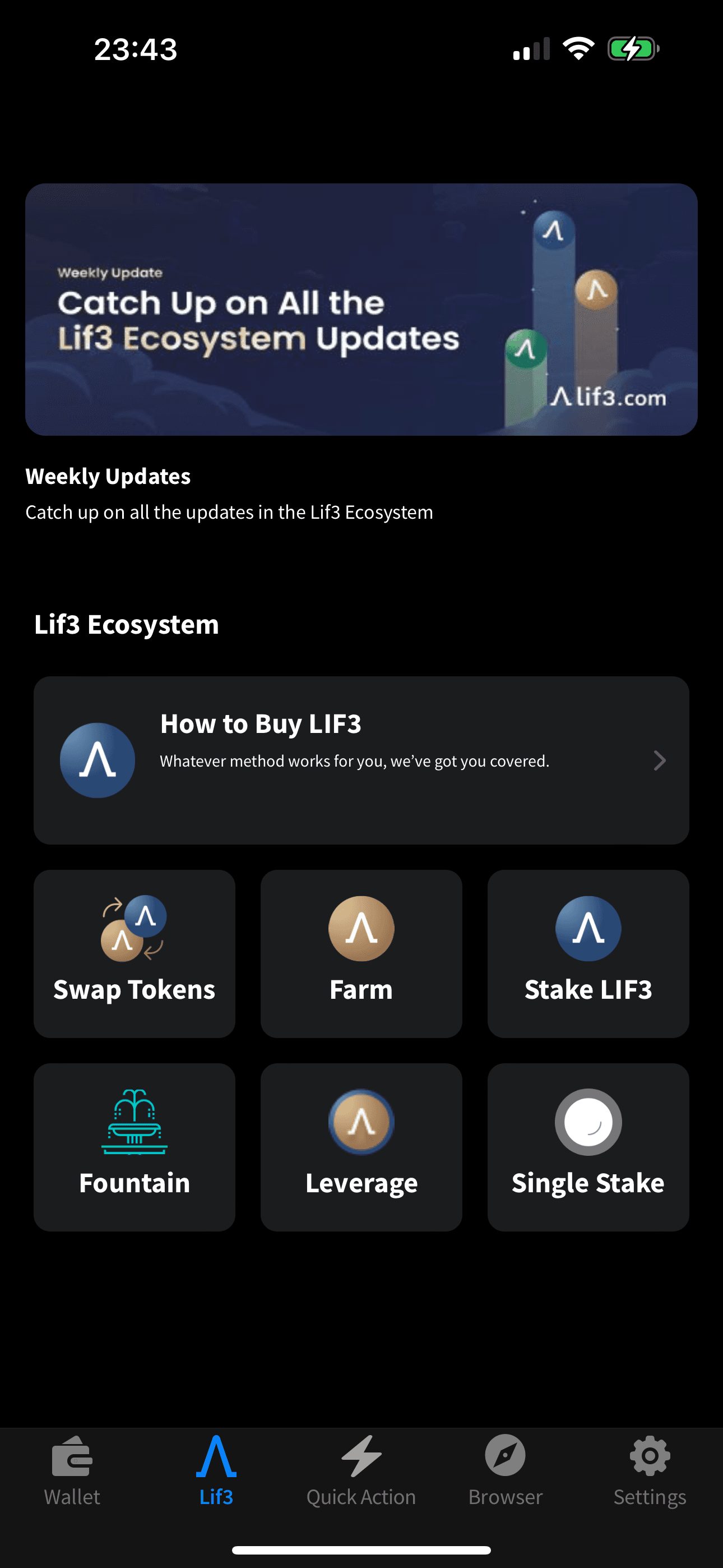A screenshot with a black background displays a digital interface at 23:43, indicating that the battery is charging. The interface promotes "Catch up on all the life ecosystem updates" and mentions the website "alif3.com" (where the '3' replaces an 'E' in "life"). The interface includes categories like "Weekly Updates", "Life Ecosystem", "How to Buy Life" and other informational sections. A prominent blue circle with an 'A' (styled without the horizontal line) appears, possibly indicating a section about swapping tokens. The interface also features six gray squares with options for "Swap Tokens," "Farm," "Stake Life," "Fountain," "Leverage," and "Single Stake." At the bottom of the screen, navigation icons include "Wallet," "Life," "Quick Action," "Browser," and "Settings," with a white bar situated centrally at the bottom.